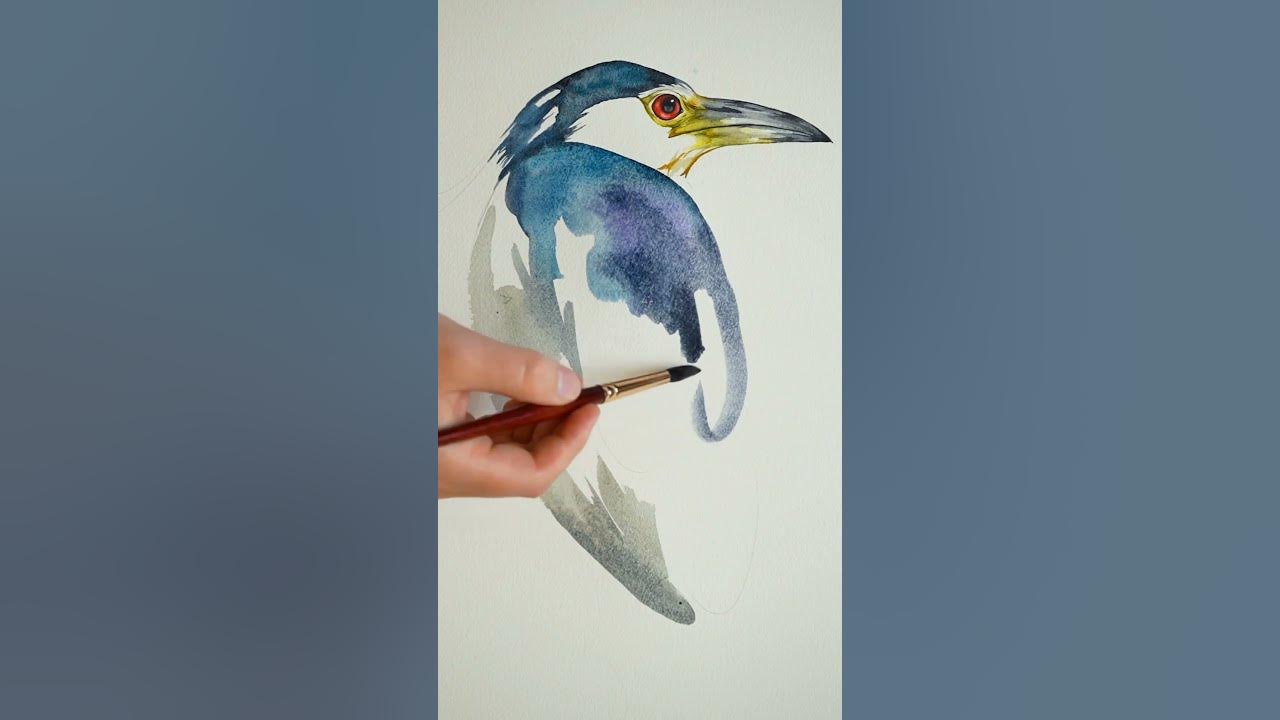The image captures an indoor scene of a partially completed watercolor painting of a bird on a horizontally rectangular piece of white paper. The painting, which appears to be on a stage for display, is encased by thick, dark gray borders on both the left and right sides. At the center of the image, the bird is in the midst of being painted, with a right hand, shown from the left of the image, holding a paintbrush delicately. The hand is Caucasian, visible from the thumb and index finger gripping a paintbrush with a brown handle, gold tip, and dark black bristles.

The bird depicted in the painting is in profile, facing right, characterized by its long, gray beak touched with a hint of yellow, striking red eye with a black pupil, and a head adorned with light blue feathers. The top half, particularly the wings, showcases a blend of blue and purple hues, transitioning to a light gray color that deepens as it extends downward. Notably, the painting is incomplete, with a large, unpainted section in the middle of the bird and parts of the wing left unfinished. The background of the canvas is painted a very light gray, providing a subdued backdrop to the vibrant colors of the bird in progress.